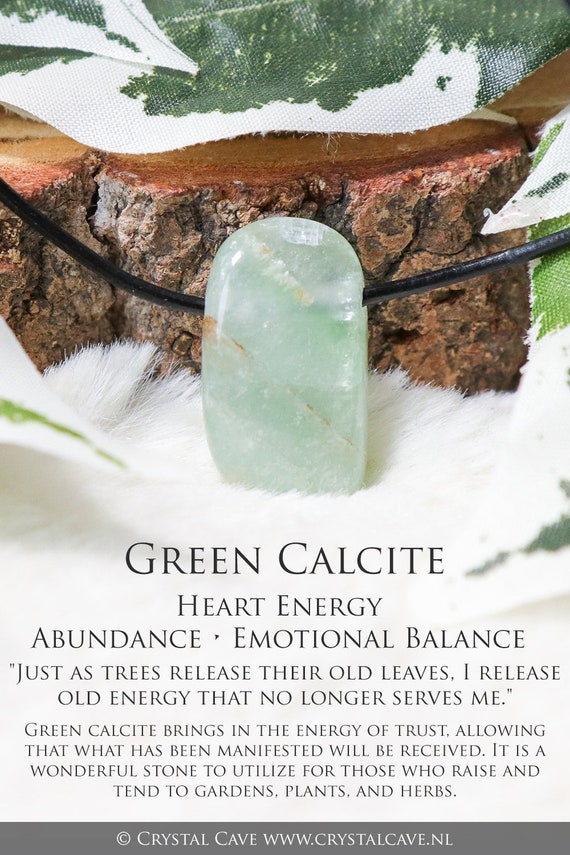The image showcases a detailed advertisement for Green Calcite, set against a visually appealing background that features a white fur-like surface and a brown driftwood or stone piece behind it, evoking a natural, rustic aesthetic. The Green Calcite crystal itself is a light green stone with intricate white veins, suspended on a string that could suggest its use as a pendant or part of a necklace. Below the crystal, text in black lettering reads: "Green Calcite - Heart Energy, Abundance, Emotional Balance. Just as trees release their old leaves, I release old energy that no longer serves me. Green Calcite brings in the energy of trust, allowing that what has been manifested will be received. It is a wonderful stone to utilize for those who raise and tend to gardens, plants, and herbs." Additionally, there is a gray stripe at the bottom indicating a copyright by Crystal Cave and their website, www.crystalcave.nl. This promotional material, likely for crystal healing enthusiasts, highlights Green Calcite's benefits and its connection to emotional release and growth.